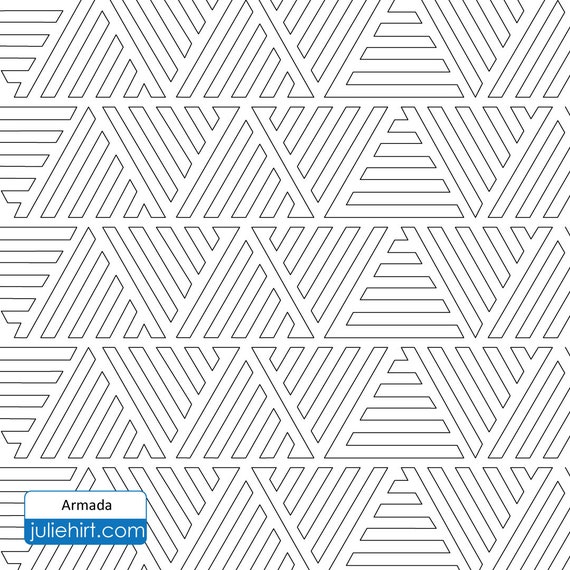The image displays an intricate black and white graphic design featuring a repeating pattern of interlocking triangles. These triangles alternate between being right side up and inverted, creating a maze-like effect with each triangle not just being outlined, but filled with additional line work. The pattern spans across eight triangles per row and forms five total rows. The corners of the design are cropped. In the bottom left-hand corner, a rectangle outlined in blue mimicks an old-fashioned peel-and-stick name tag. The upper half of this rectangle is filled with white and contains black text that reads "Armada," while the bottom half is filled with blue and displays white text that says "juliehirt.com" (Hirt spelled H-I-R-T). This part of the image seems to indicate the name of the artist and her website. Overall, the design is angular, clean, and appears to have been created using computer software.